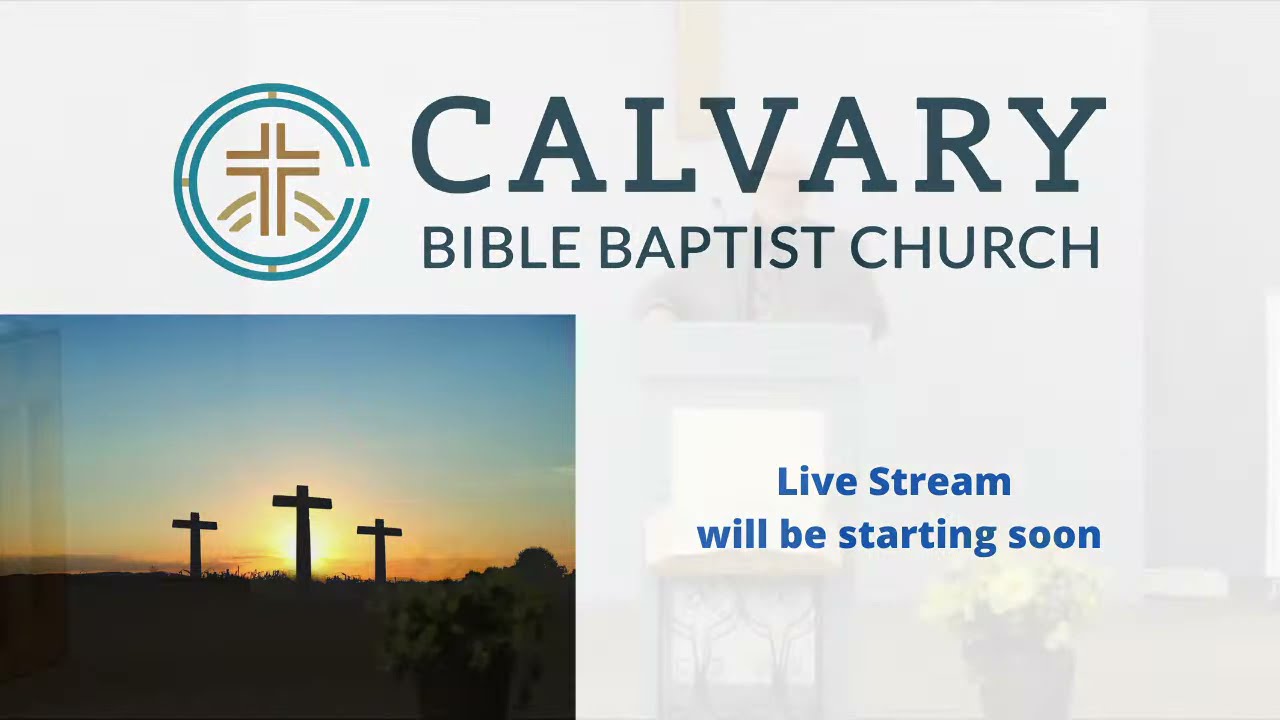The image appears to be an advertisement for Calvary Bible Baptist Church, featuring elements that suggest it is a live stream announcement. The background is predominantly white, providing a clean canvas for the content. At the top of the image, the text "CALVARY" is prominently displayed in large, all-capitalized dark blue letters. Beneath that, in a smaller font but still in all capitals, are the words "BIBLE BAPTIST CHURCH."

To the left of the text is the church's logo, which comprises a circular or C-shaped blue design with a gold cross at the center, flanked by two golden arches on either side. This logo ties the religious symbolism neatly with the text.

In the lower left corner of the image, there’s a visually evocative scene of a field with three crosses mounted on a hill, set against a backdrop where the sun is either setting or rising. The sky transitions from a deep blue to a warm orange hue as it nears the horizon, highlighting the central cross.

Additionally, in the bottom right corner of the image, there's text in blue indicating "LIVE STREAM, WE'LL BE STARTING SOON," suggesting an imminent online service or event. This digital cue implies that the content might be available on a platform such as YouTube or directly on the church’s website. The careful arrangement of these elements creates a cohesive and descriptive advertisement for the church’s live streaming service.